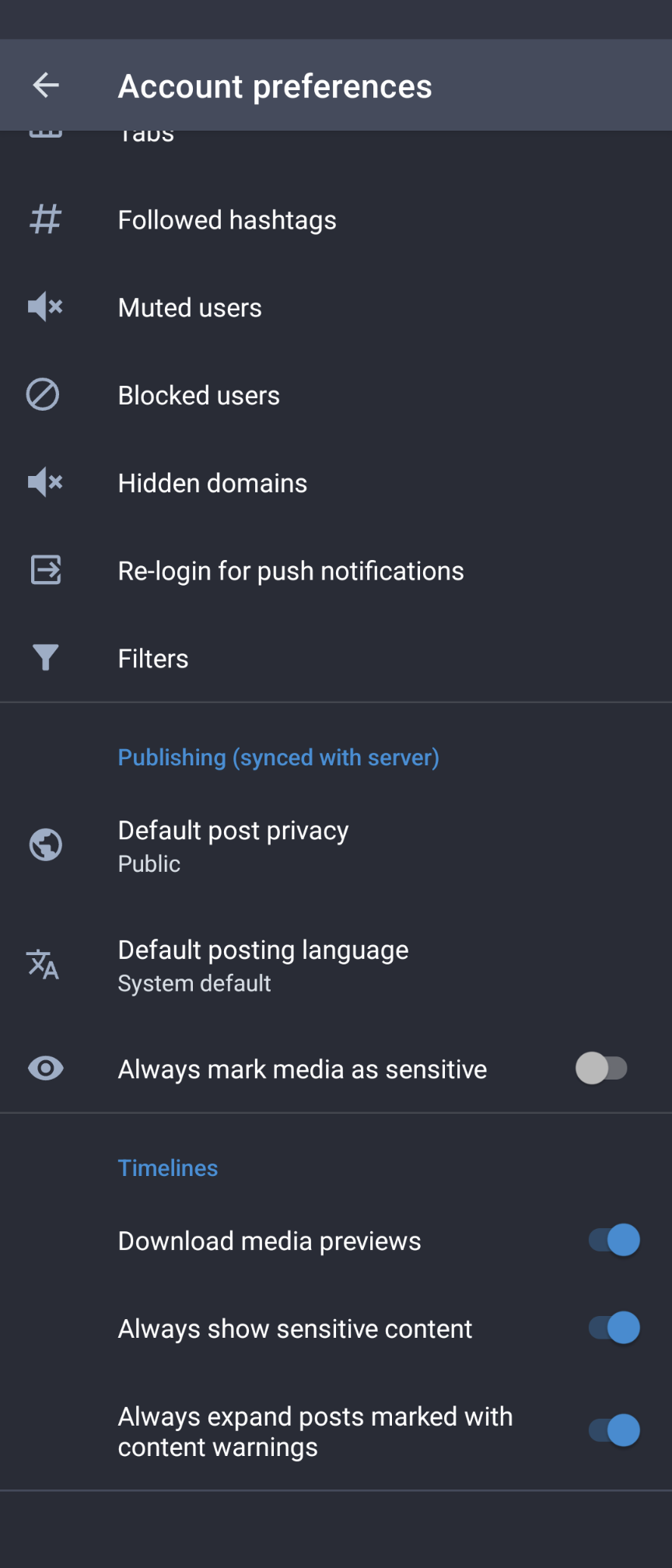**Detailed Caption:**

A screenshot captured from a mobile device showcasing an application interface with a predominantly black background and contrasting white text. There are elements of blue text incorporated throughout the interface. 

At the top of the screen, a banner with a gray background features white text that reads "Account Preferences." Adjacent to this, on the left, is a white arrow icon pointing to the left. Below the banner, the word "Tabs" appears in white text.

The interface includes several sections:
1. "Followed Hashtags" - marked by a hashtag symbol, displayed in white text.
2. "Muted Users" - denoted by a speaker icon with an X, also in white.
3. "Blocked Users" - represented by a circle with a line through it, in white.
4. "Hidden Domains" - indicated with a speaker icon and an X, similar to Muted Users.

Below these sections, there is a right-arrow icon encased in a square, indicating the option to "Re-Login for Push Notifications."

Further down the screen, in blue text, the following settings are detailed:
- "Published: Synced with server."
- "Default Post Privacy: Public" accompanied by a globe icon.
- "Default Posting Language: System Default."

Additionally, there is an "i" icon paired with the option labeled, "Always Mark Media as Sensitive."